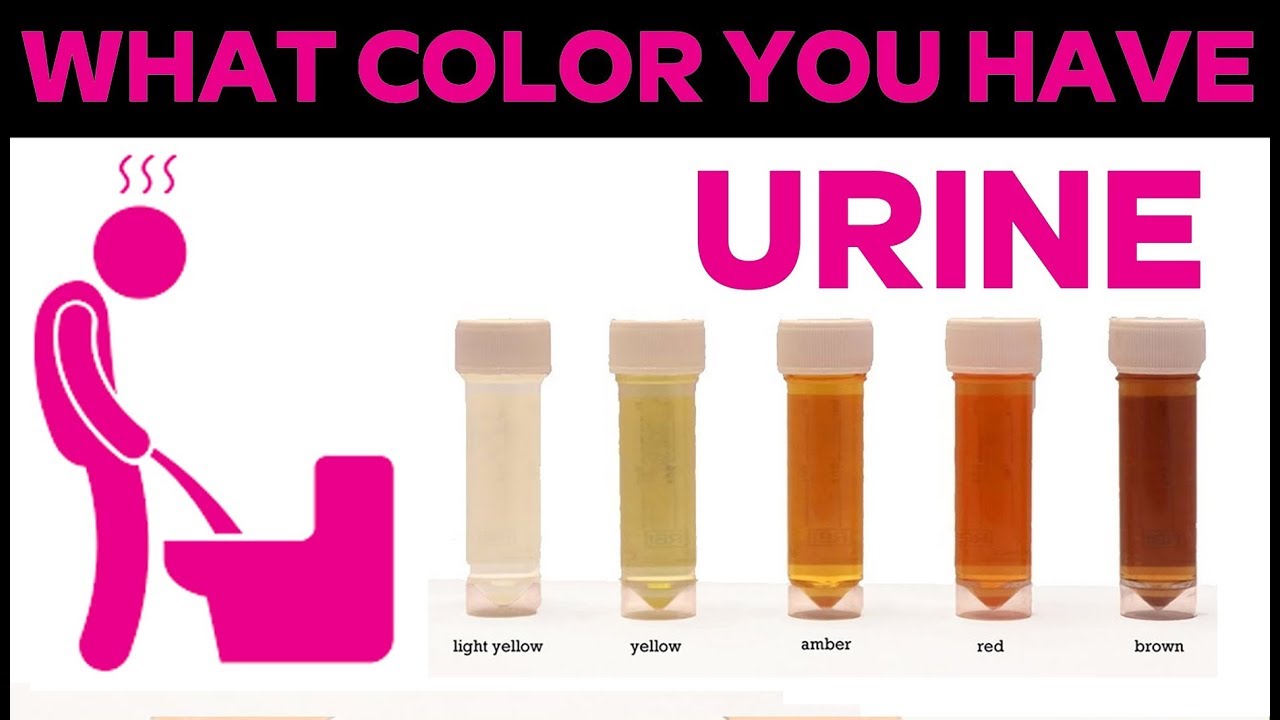The infographic features a sleek design with a clear white background accented by a thick black border at the top, where large, bold, pink text declares, "WHAT COLOR YOU HAVE." Below this heading, on the white background, a stylized, pink-colored stick-figure man is depicted urinating into a toilet, with wavy lines above his head suggesting confusion. To the right of this figure, in the upper right corner, bold, pink text labels the visual as "URINE."

In the forefront of the infographic, five transparent plastic vials with white, ribbed caps are neatly arranged from left to right. Each vial displays a different color of urine, progressing in shade from left to right. Beneath each vial is a label indicating the corresponding color:
- The first vial contains a very light yellow, almost clear, labeled "light yellow."
- The second vial is a slightly darker shade, labeled "yellow."
- The third vial displays a light orange hue, labeled "amber."
- The fourth vial holds a darker, orange-red liquid labeled "red."
- The fifth and final vial shows a brown color, labeled "brown."

This detailed infographic effectively conveys the various colors of urine and their corresponding descriptions.